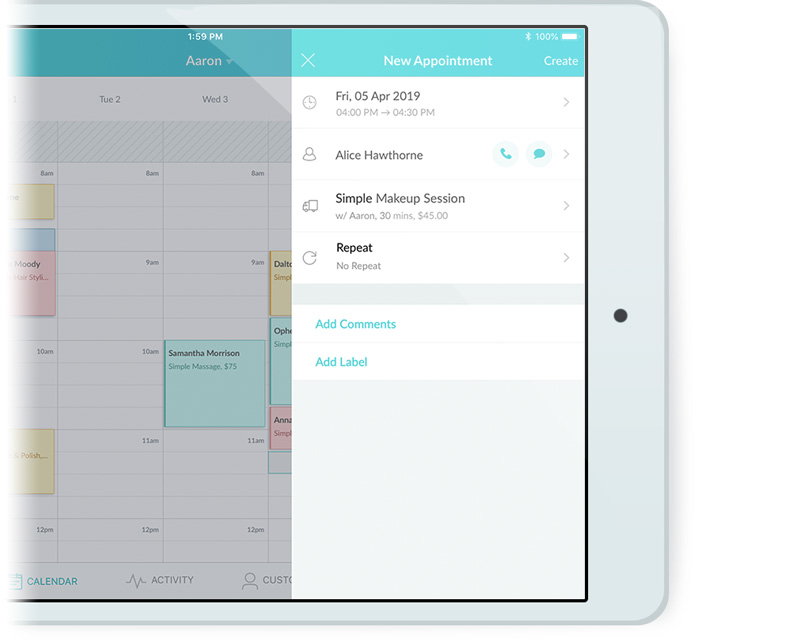The image features the right half of an iPad screen displaying a calendar application open to Friday, April 5th, 2019. Highlighted on the screen is an appointment for Alice Hawthorne, marked as a "simple make-up session" with options to add comments and labels, and no repeat set. The calendar's header is in light blue, while the main body is predominantly white, with appointments color-coded in red, yellow, and light blue.

The composition appears professionally crafted, likely for advertising purposes. The left side of the image, where the iPad ends, is intentionally washed out, suggesting a high-quality brochure or website display to showcase the device in action. This artistic choice highlights the functionality of the calendar app while drawing attention to the sleek design of the iPad.